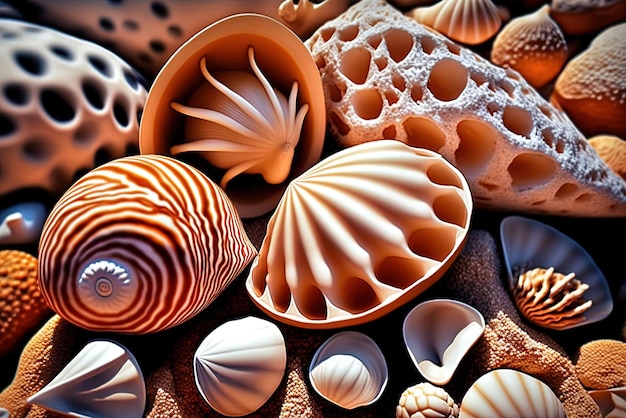This digital image captures an array of seashells laid out in a visually appealing and organized manner, resting on a surface that seems to be either a blanket, towel, or possibly brown sand. The seashells vary greatly in shape and size, including some with distinctive spiral patterns and others more reminiscent of clams, alongside coral-like structures with characteristic holes and dimples. The image palette is tightly coordinated, dominated by shades of pink, white, and various hues of brown and beige. Notably, a large shell on the left side features striking orangish-white concentric lines, and next to it, a slightly opened shell appears to contain a small, spherical object with tendrils extending back into the shell, contributing to the overall alien, slightly surreal appearance of the scene.